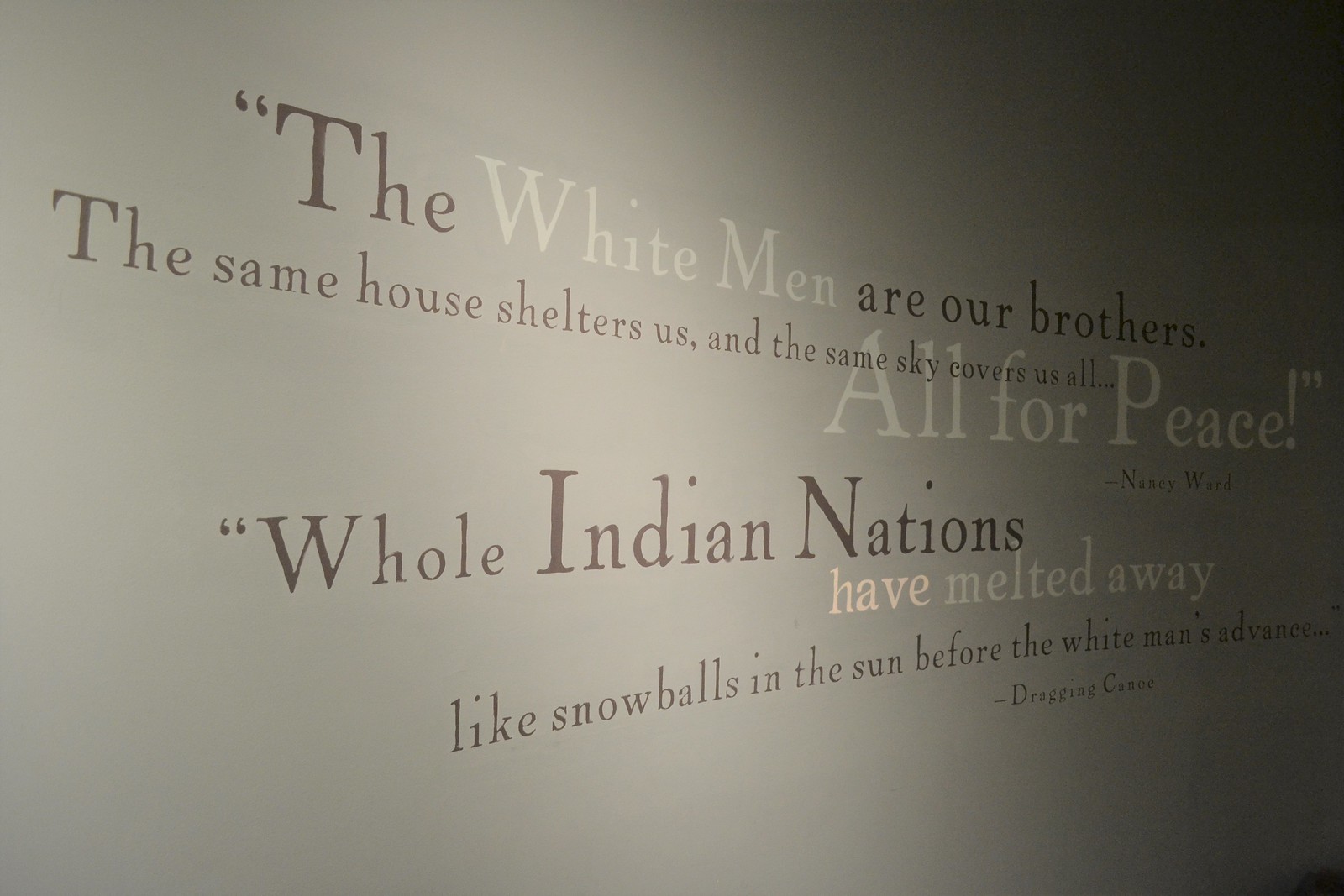This photograph depicts a gray-painted wall featuring two quotations in black and white text. The first quotation, attributed to Nancy Ward, reads, "The white men are our brothers. The same house shelters us and the same sky covers us all. All for peace!" This text is predominantly in black. Nancy Ward's name is spelled "W-E-R-D" in the caption. The second quotation, by Dragging Canoe, states, "All Indian nations have melted away like snowballs in the sun before the white man's advance." In this quote, the phrase "melted away" is highlighted in white, with the remainder of the text in black. The right side of the image appears somewhat darkened, while the left side is brightly illuminated.